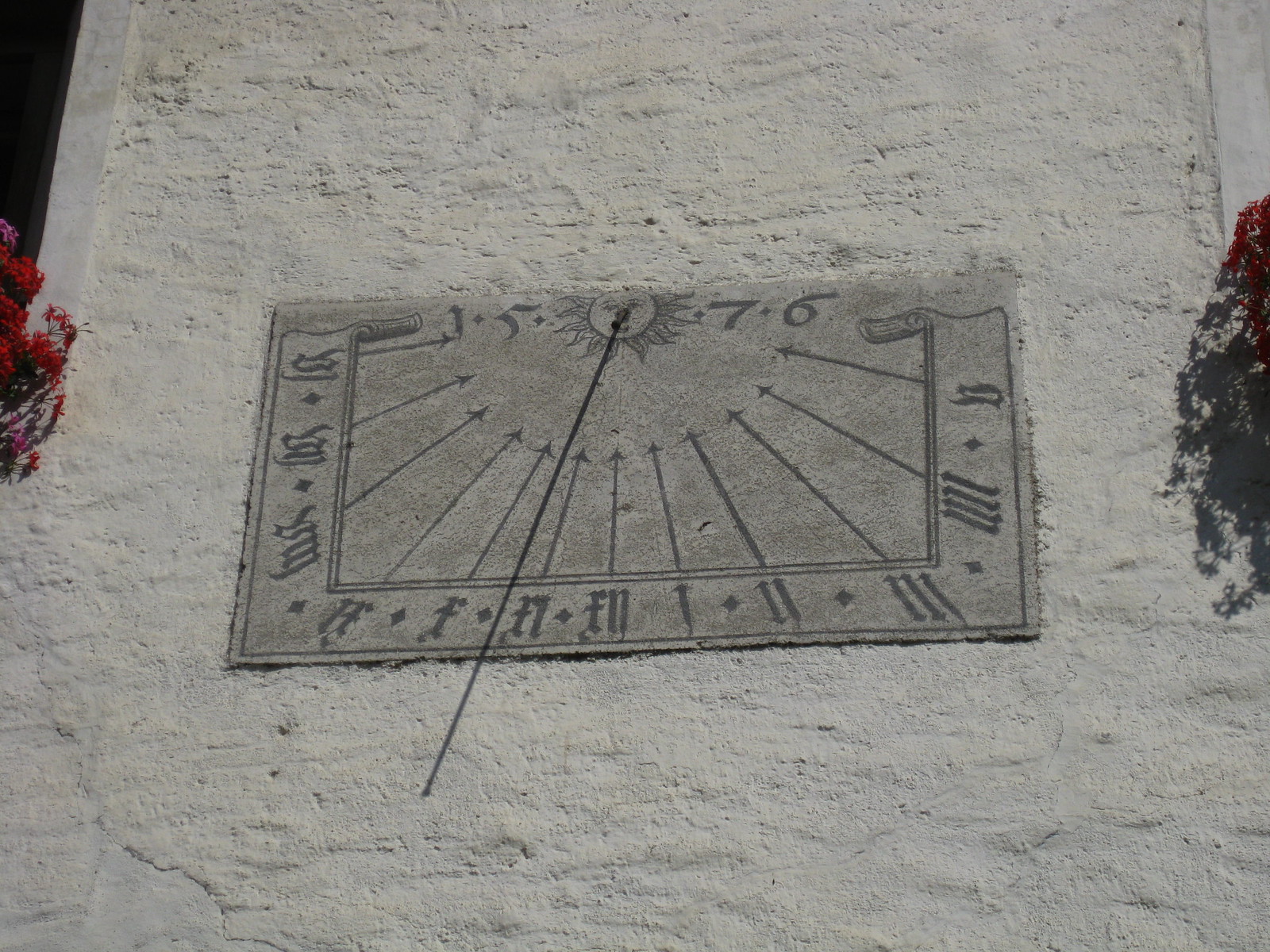In this close-up image, the focal point is a square-shaped, gray sundial-like object positioned at the center. The sundial is surrounded by a textured, light gray stone, giving an ancient and weathered appearance. To add a touch of natural beauty, red flowers can be seen on both sides of the sundial; on the left side, a prominent cluster of red flowers is visible, while on the right side, a smaller portion of red flowers appears with a shadow underneath, casting a dark gray tone. The majority of the background is occupied by this gray stone, creating a solid yet intricate visual. In the top left corner, a small section of the background appears black, contrasting with the stone. The sundial itself features a central point where multiple arrows converge. At the top, there is an inscription with the numbers "15" to the left and "76" to the right, alongside Roman numerals that trace the sundial's outer edges. A distinct black hand extends towards the left portion of the sundial, adding an element of functionality to this historical timekeeping device.